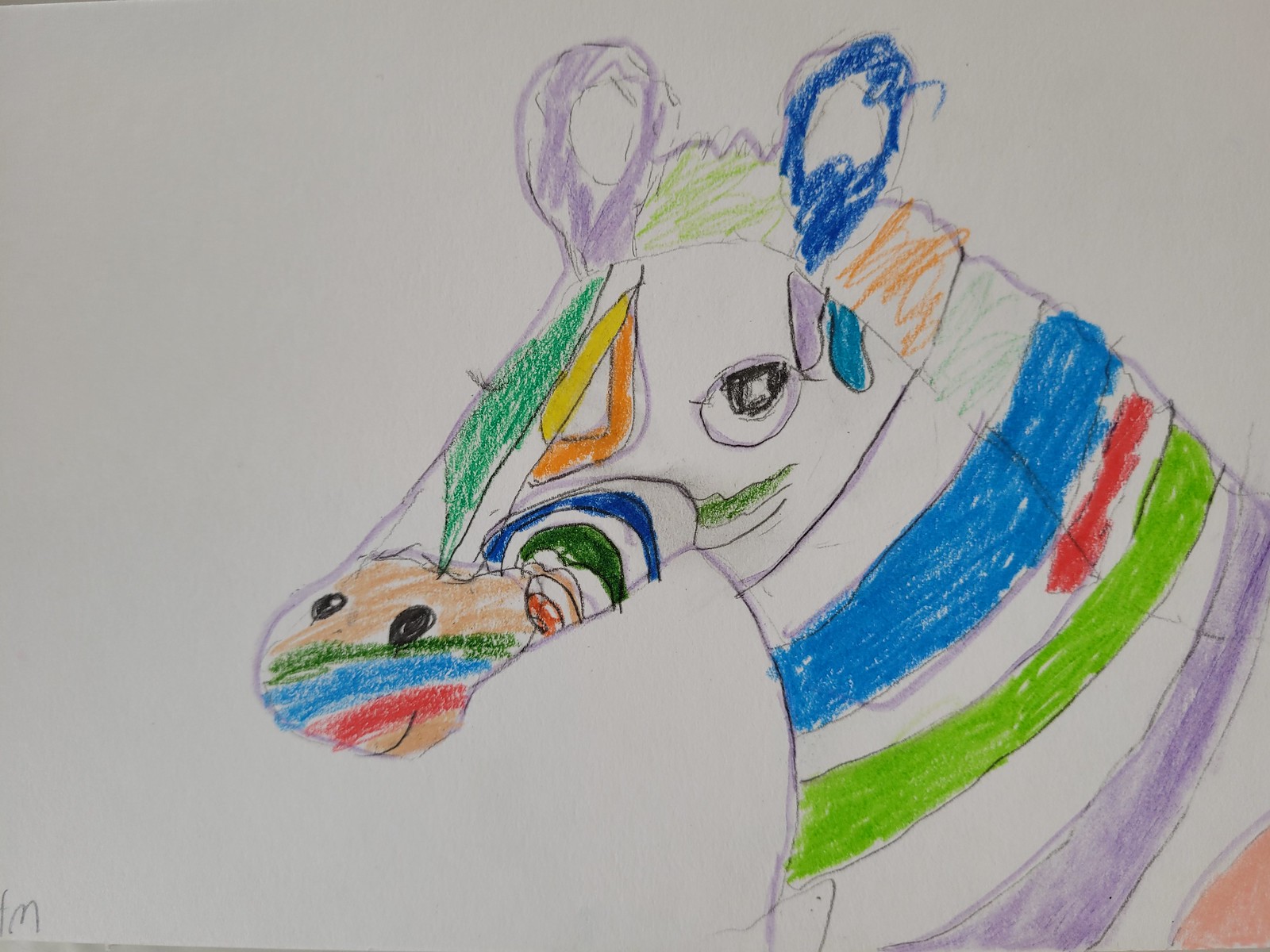The image is a playful and colorful children's drawing of a zebra-like animal, prominently featuring its whimsically striped head in the center. The animal's nose is tilted downwards towards the bottom left corner, with an arrangement of vibrant, multicolored stripes adorning its face, running from peach and purple to green, red, blue, orange, and yellow, including varying shades of green. The drawing appears to be outlined in a dark pencil, with certain sections retraced for added emphasis, creating a slightly darker contour. The zebra-like creature sports a cheerful smile, two distinct nostrils, a large expressive eye, and two ears—one purple and one blue—along with a mane. Below its nose, a smaller section features additional stripes. The entire artwork is rendered on a white piece of paper, with the small letter "M" inscribed in pencil in the bottom left corner, potentially signifying the artist's initial or a signature. The colors used appear to be filled in with oil pastels or colored pencils, adding a rich texture to the drawing.